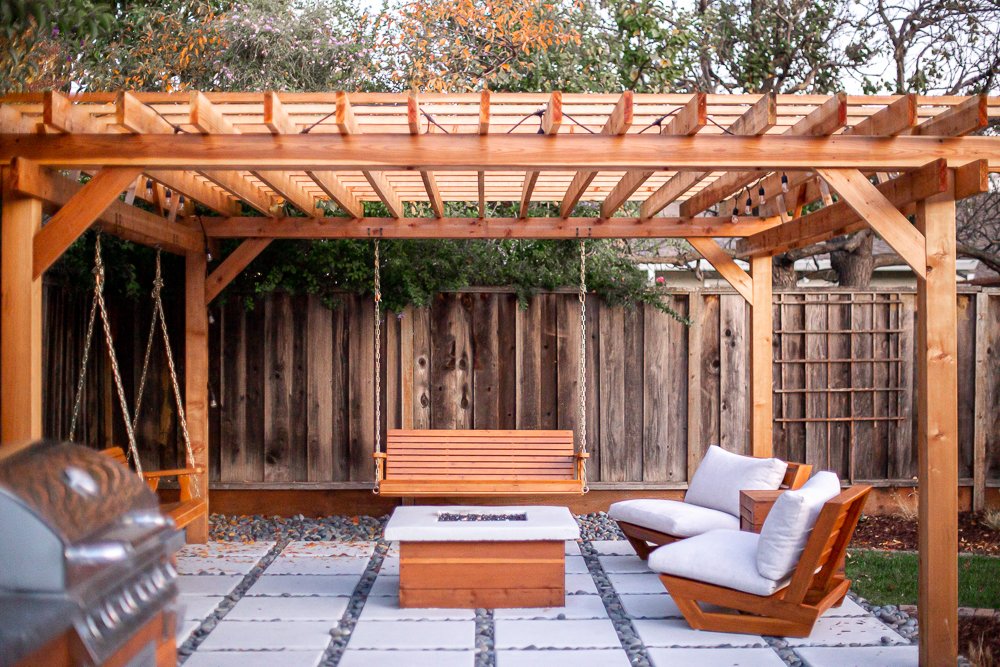This photograph showcases a beautiful backyard patio area covered by a large, rustic wooden pergola with an open roof. The square patio is marked out by white tiles laid atop a gravel base, creating a defined and clean space in the middle of the yard. Central to the patio is a sophisticated wooden table with a white marble top, likely functioning as a fire pit, accented by a distinctive black center where flames can be seen.

Suspended from the pergola are two large, inviting wooden benches, each designed to swing gently. To the right of the seating area are two wooden chairs with plush white cushions, providing additional comfort around the fire pit. Notably, the seating structures and the furniture exhibit a rich reddish-brown hue, injecting warmth into the space.

In the foreground, on the left side, a high-end barbecue grill stands ready for use, its silver top gleaming. The entire area is bordered by a tall, sturdy wooden fence, notably grayish-brown, which adds a rustic charm and offers a sense of privacy. Behind the fence, lush trees can be seen, adding a touch of nature and greenery. A small patch of grass can be observed to the right side of the patio, blending seamlessly with the white tiles and gravel. The meticulous arrangement of elements within this photograph highlights a perfect blend of function and style in an outdoor retreat.